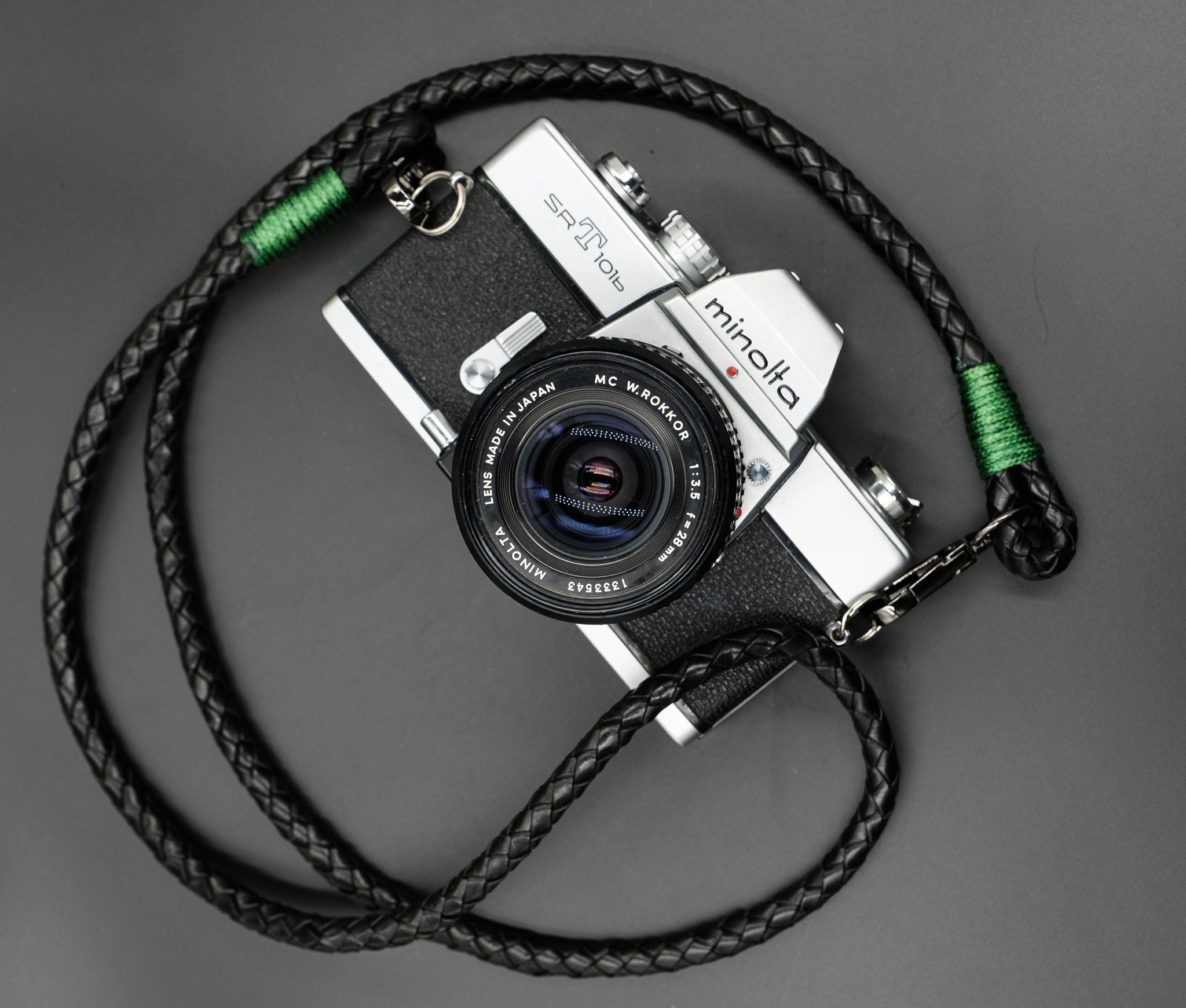This photograph captures a detailed, angled view of a black and silver Minolta SRT 101 camera, showcasing its vintage yet refined appearance. The camera features an adjustable lens prominently branded with "Made in Japan," further highlighting its classic build. Accompanying the camera is a high-quality, artistic braided leather strap with distinctive green accents. The strap intricately wraps around the camera, joined at metal loops on either side, suggesting both functionality and style. The overall presentation evokes a sense of nostalgic elegance, making one ponder whether it's a meticulously refurbished film camera or a stylized digital version.